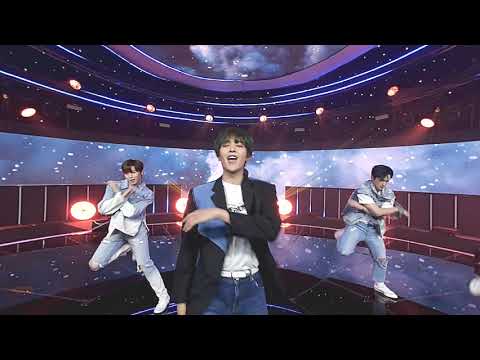The image is a vibrant color photograph of a performance by a Korean boy band on a futuristic, spaceship-themed stage. At the center, the lead singer stands out, wearing a dark jacket with a blue sash on one side, a white t-shirt, blue jeans, and a white belt. His arm is poised at chest height, emphasizing his singing. Behind him, two dancers with similar hairstyles that are dark and straight, are energetically dancing with one leg raised and arms crossed at chest level. Both dancers wear ripped blue jeans, white shoes, and blue jean jackets; the one on the right sports a short-sleeved jacket over a white t-shirt, while the one on the left has long sleeves. The stage backdrop features a space theme, adorned with stars and cosmic clouds, enhanced by spotlights that add to the dynamic atmosphere.